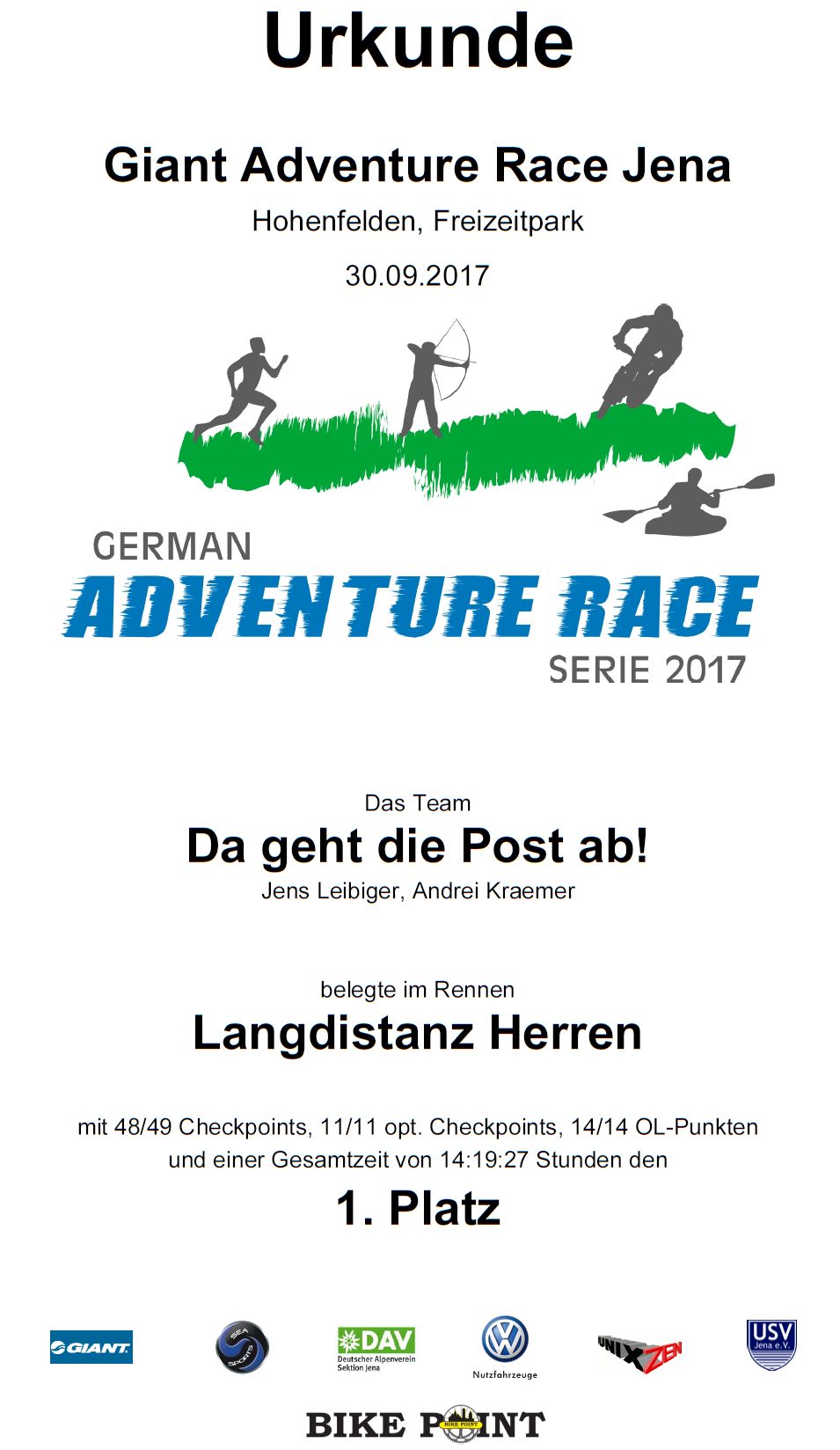This advertisement is a vertical, rectangular, white-background graphic for the "URKUND Giant Adventure Race Jena Hohenfelden Freisel Park," scheduled for September 30, 2017. The ad features a series of digital silhouettes depicting individuals engaging in various outdoor activities on green grass: a man running, a person shooting a bow and arrow, a cyclist, and a kayaker. The German Adventure Race Series 2017 is prominently displayed in blue text, beneath which it further details the team—Jens Leibinger and Andre Kramer—and mentions the event includes 48/49 checkpoints and 11/11 optional checkpoints, summing up to a total time of 14:19:27. At the bottom of the advertisement, there are six sponsor logos, including recognizable brands such as Giant, DAV, Volkswagen, and USB, along with a logo reading "Bike Point."